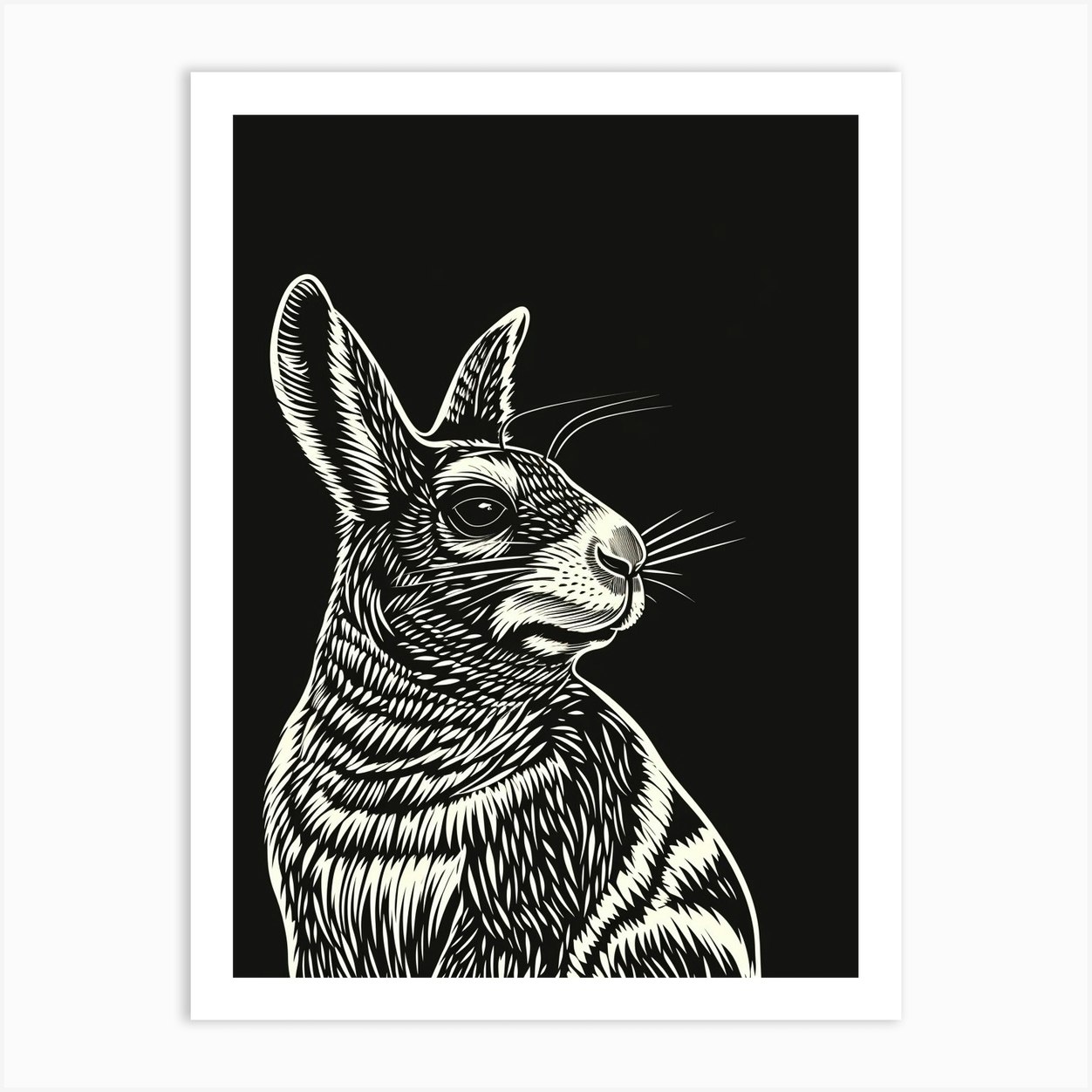This vertically oriented photograph appears to be a meticulously crafted black and white artwork with a white frame. The main focus of the image is a highly detailed, artistic sketch of a rabbit, rendered entirely in white on a flat black background. The rabbit, which occupies roughly the top three-quarters of the frame, is depicted with delicate white brush strokes that vividly bring out its features, from its very long whiskers to the V-shaped ears and attentive gaze. The stark contrast between the white details of the sketch and the black background enhances the rabbit's lifelike appearance, as if it was painted directly onto the black surface. The rabbit is oriented to the right, giving the impression of it being alert and observant. This could be a photograph of an actual hand-drawn illustration or a digitally created piece, but either way, it captures the realistic essence of a rabbit in the wild through a monochromatic theme with no additional colors or text.